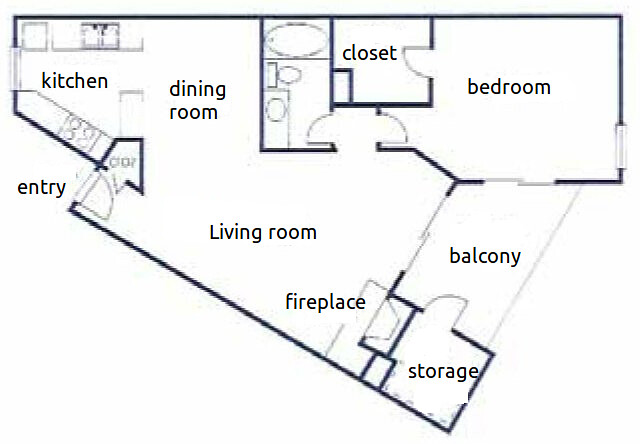This digital illustration depicts a detailed floor plan of a modest-sized apartment. The layout is thoughtfully designed and clearly labeled with text indicating the function of each room. The overall shape of the floor plan is rectangular, but the lower half inclines diagonally, creating an uneven diamond shape.

In the top-left portion of the image, the floor plan starts with the kitchen, which includes key appliances like a sink, refrigerator, and stove. Adjacent to the kitchen is the dining room. You enter the apartment through an entryway located below the kitchen; turning left from the entryway leads you into the dining room and then into the kitchen. The kitchen also features a window.

Below the dining room, continuing from the entryway, is the living room, which is equipped with a fireplace. To the left of the living room, there is a bathroom, and directly across from it is the bedroom, complete with a closet.

Additional features of the apartment include a balcony located below the bedroom and extra storage space situated behind the fireplace in the living room. Overall, the floor plan presents a well-organized and efficiently utilized space, perfect for comfortable living.